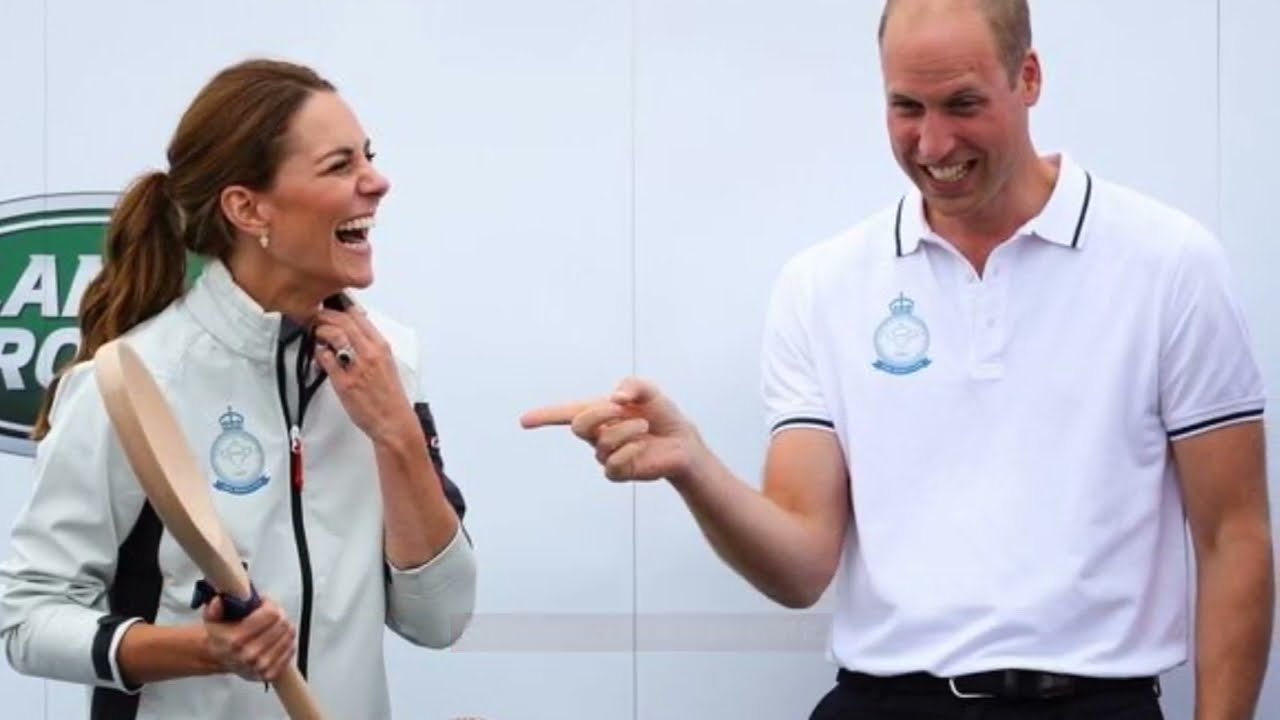The photograph captures Prince William and his wife Catherine, both engaged in a delightful moment of laughter. Catherine, positioned on the left, holds a wooden paddle shaped like a tennis racket. She dons a white sports jacket with a black zipper in the front and black accents on the sleeves, her long brown hair is tied back in a ponytail. Notably, she clutches her jacket's collar with her right hand. Prince William stands slightly to the right, laughing and pointing a finger at her, seemingly engrossed in their humorous exchange. He wears a white short-sleeved shirt, identical in emblem to Catherine's, paired with black trousers and a belt. They are positioned against a white wall that prominently displays a logo, likely Land Rover, featuring a green and white oval. The scene appears to be set outdoors, possibly during an event on a bright day, encapsulating a genuine moment of joy between the couple.